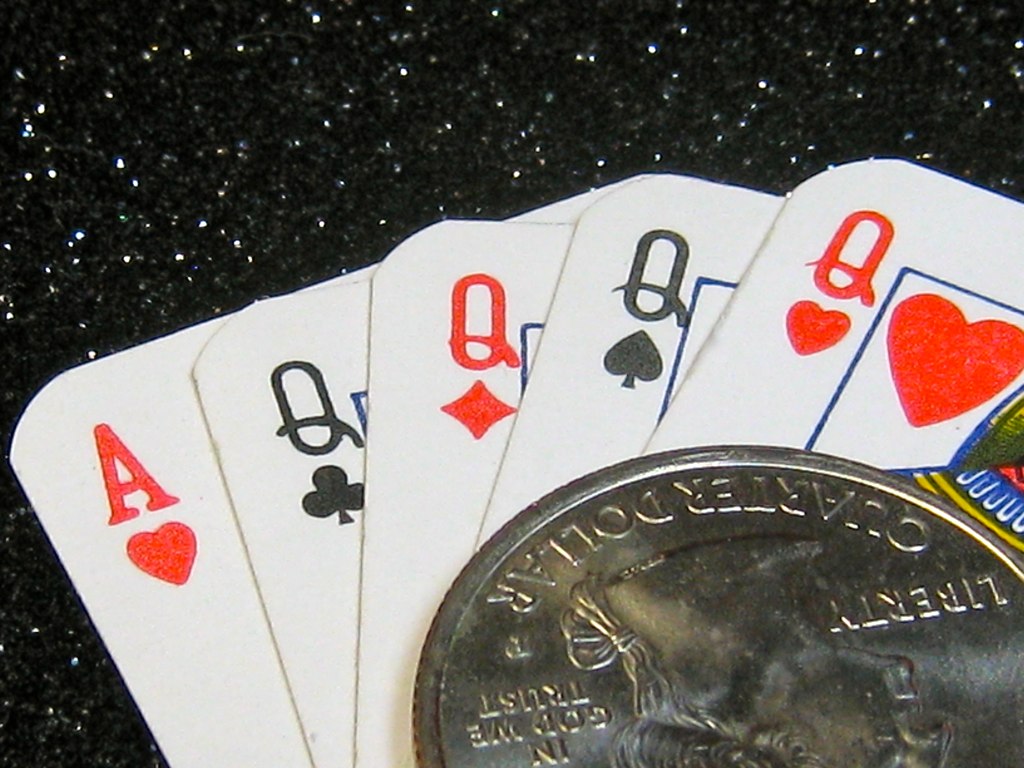An up-close view showcases five playing cards laid out on a glimmering black background adorned with silver glitter, creating a striking contrast. The cards are spread in a fan-like arrangement, revealing their faces. The lineup includes the red Ace of Hearts, the black Queen of Clubs, the red Queen of Diamonds, the black Queen of Spades, and the red Queen of Hearts. A quarter, displaying the inscriptions "Quarter Dollar," "Liberty," and "In God We Trust" along with a detailed side profile of George Washington, rests partially over three of the cards, adding a touch of intrigue to the scene. This meticulously arranged composition creates a visually captivating tableau.